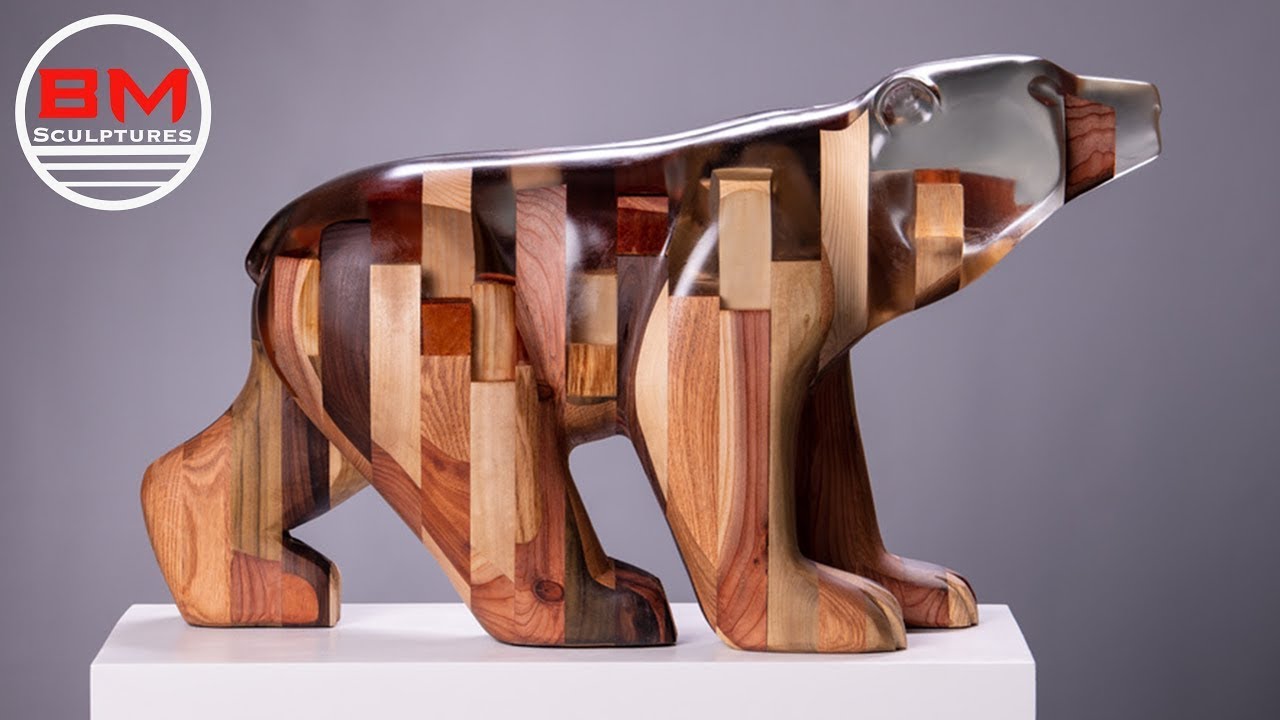This photograph captures a meticulously crafted sculpture of a polar bear, prominently displayed on a white pedestal against a gray backdrop. The bear, seen in profile, is made from various types of polished wood, each piece showcasing different shades and grains, arranged in an irregular but harmonious pattern. The detailed woodwork covers the bear's body, while its head transitions into a clear, glass-like material, except for the nose, which retains a streak of wood. The bear appears to be in mid-stride, with one back foot forward and its two front paws placed together on the pedestal. The top left corner of the image features the logo "BM Sculptures" in red and white, encircled by a white border, with three underlines beneath the word "Sculptures."